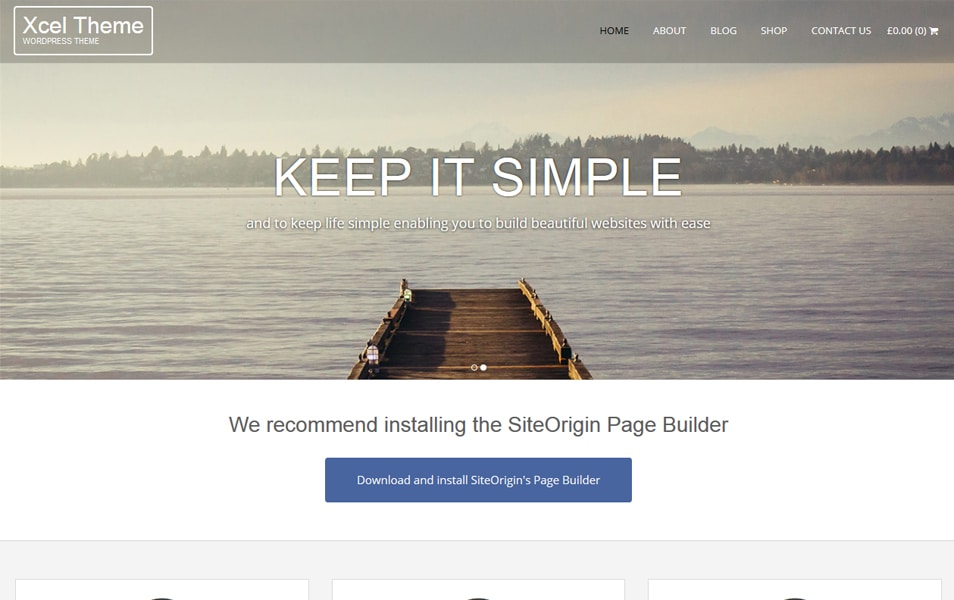The image displays a section of a website with a taupe gray background at the top. On the top left, there is a white outline with the text "ExcelTheme" in white capital and lowercase letters, indicating a WordPress theme. Moving to the right, there are navigation links in black print: "Home," "About," "Blog," "Shop," and "Contact Us." Next to these links, it shows a monetary value of "£0.00" with "zero" in parentheses, followed by a shopping cart icon.

Below this, there is a large graphic that appears to be an outdoor scene. Although the graphic is slightly muted, it depicts a sky with scattered clouds, transitioning down to a landscape featuring trees and mountains in the distance. Beneath this landscape, a body of water is visible, with a wooden dock extending into it from the center. The dock is simple, with no railings.

Centered on the image, a bold white text in capital letters reads, "KEEP IT SIMPLE." Underneath this, a smaller white text says, "Keep life simple by enabling you to build beautiful websites with ease."

Further down, there is a white banner with a recommendation to "install the SiteOrigin Page Builder." "SiteOrigin" is written as one word with a capital "S" and "O." Below this, a blue banner displays the text, "Download and Install SiteOrigin's Page Builder," in white.

This descriptive caption provides a detailed overview of the website's layout, graphics, and key messages.